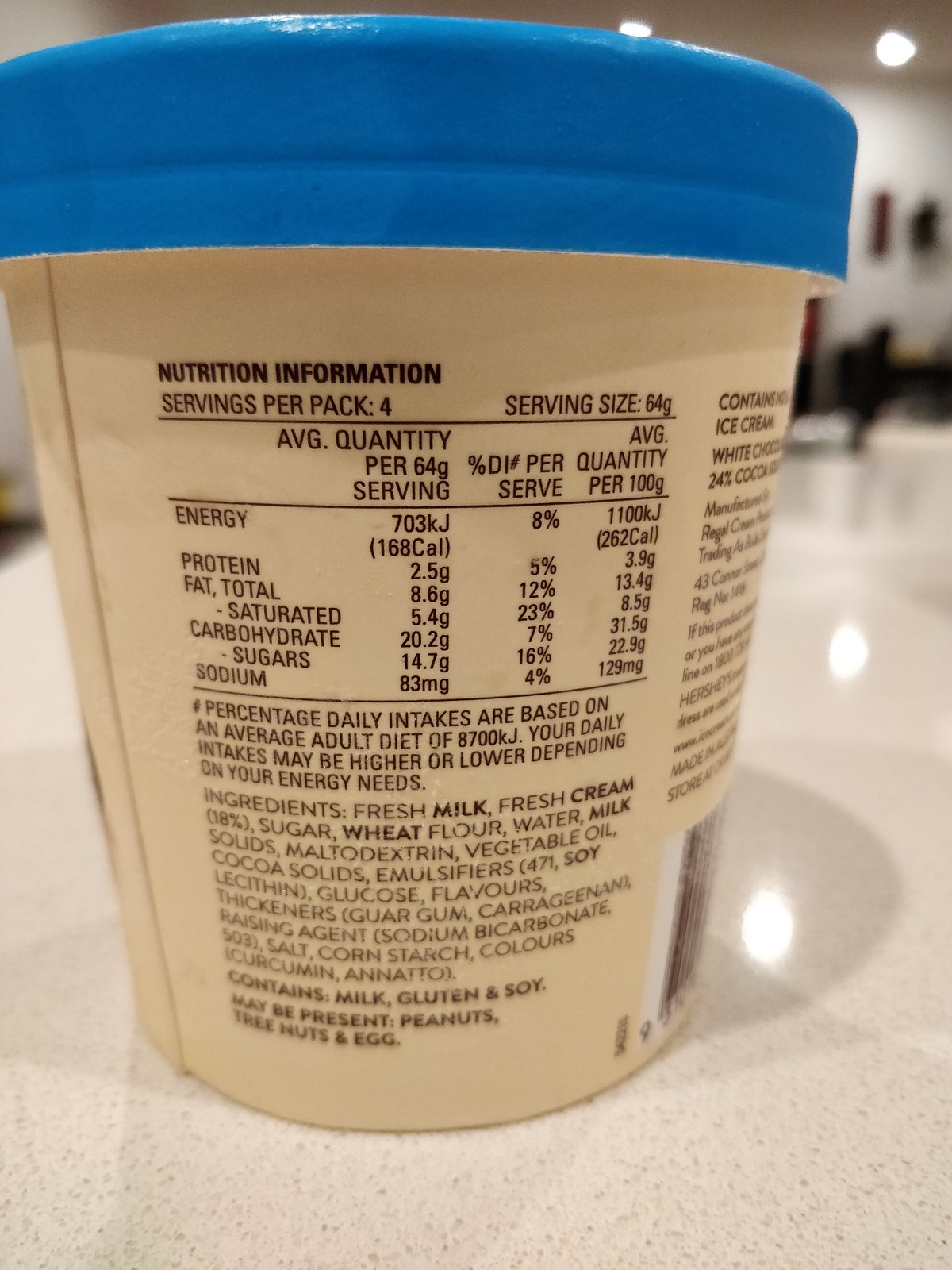In the image, we see an interior close-up of a pint-sized ice cream container placed on a light beige countertop adorned with brown and black speckles. The container has a medium tan main body with a dark blue lid, which features an indentation line around its middle. The background of the image is out of focus, showing parts of a white wall and indistinct objects, perhaps seats, hanging on the wall.

The main focus of the picture is the side of the container displaying the nutritional information. The nutritional label, written in dark brown text, details servings per pack (four), serving size (64g), and various nutritional elements including energy, protein, total fat, saturated fat, carbohydrates, sugars, and sodium. The daily intake percentages are based on an average adult diet of 8700kJ. The container also lists ingredients like fresh milk, fresh cream, sugar, wheat flour, water, milk solids, vegetable oil, and cocoa solids. It includes dietary warnings indicating the presence of milk, gluten, and soy, and possible traces of peanuts, tree nuts, and egg. Additionally, the countertop has bright white circular glares from the overhead lights, adding a reflective element to the scene.